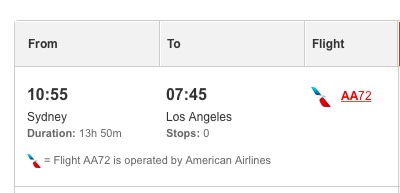A photograph captures a detailed segment of a flight itinerary, likely sourced from a travel booking website or an airport departure board. The itinerary displays a direct, non-stop flight operated by American Airlines with the flight number AA-72, symbolized by a small American Eagle emblem.

The journey originates from Sydney, Australia. The departure time is listed as 10:55, though the time of day (AM or PM) is not specified. This long-haul flight spans an impressive duration of 13 hours and 50 minutes, landing in Los Angeles, USA, at 07:45 (again, with no specification of AM or PM). This flight path demonstrates a significant traversal through multiple time zones, contributing to the apparent discrepancy between the departure and arrival times.

Overall, the documentation underscores the extensive nature of the transpacific flight connecting two major international cities without any intermediate stops.